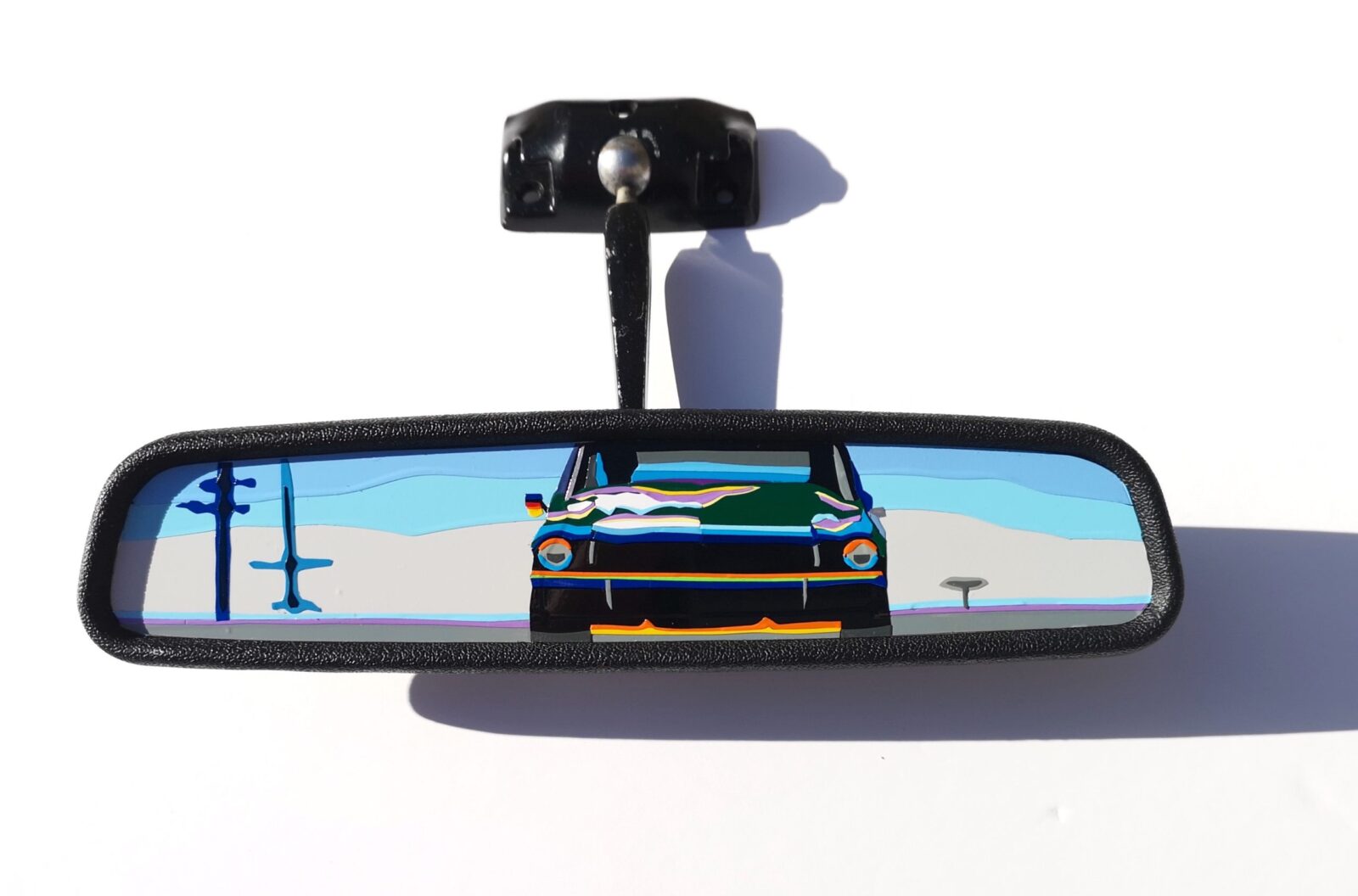The image features a black rearview mirror affixed to a white wall, casting a shadow behind it due to a light source angled from the left. The mirror, which is long and rectangular with a black handle, presents an intriguing illustration instead of a typical reflection. Within the mirror, a stylized cartoon graphic depicts a classic vehicle with round headlights. The car is predominantly green with yellow and pink accents and seats, and it is driven by a black silhouette figure. The backdrop within the mirror illustration showcases a whimsical desert-like scene with a blue, squiggly sky, transitioning from darker to lighter blue and fading into white. Below this, the ground appears greyish with a pink line. On the left side of the mirror are two street poles or electrical poles, while on the right side, there's a deserty-looking tree. The entire image within the mirror combines elements of both realism and animated artistry, with neon colors and shadow effects contributing to its unique composition.